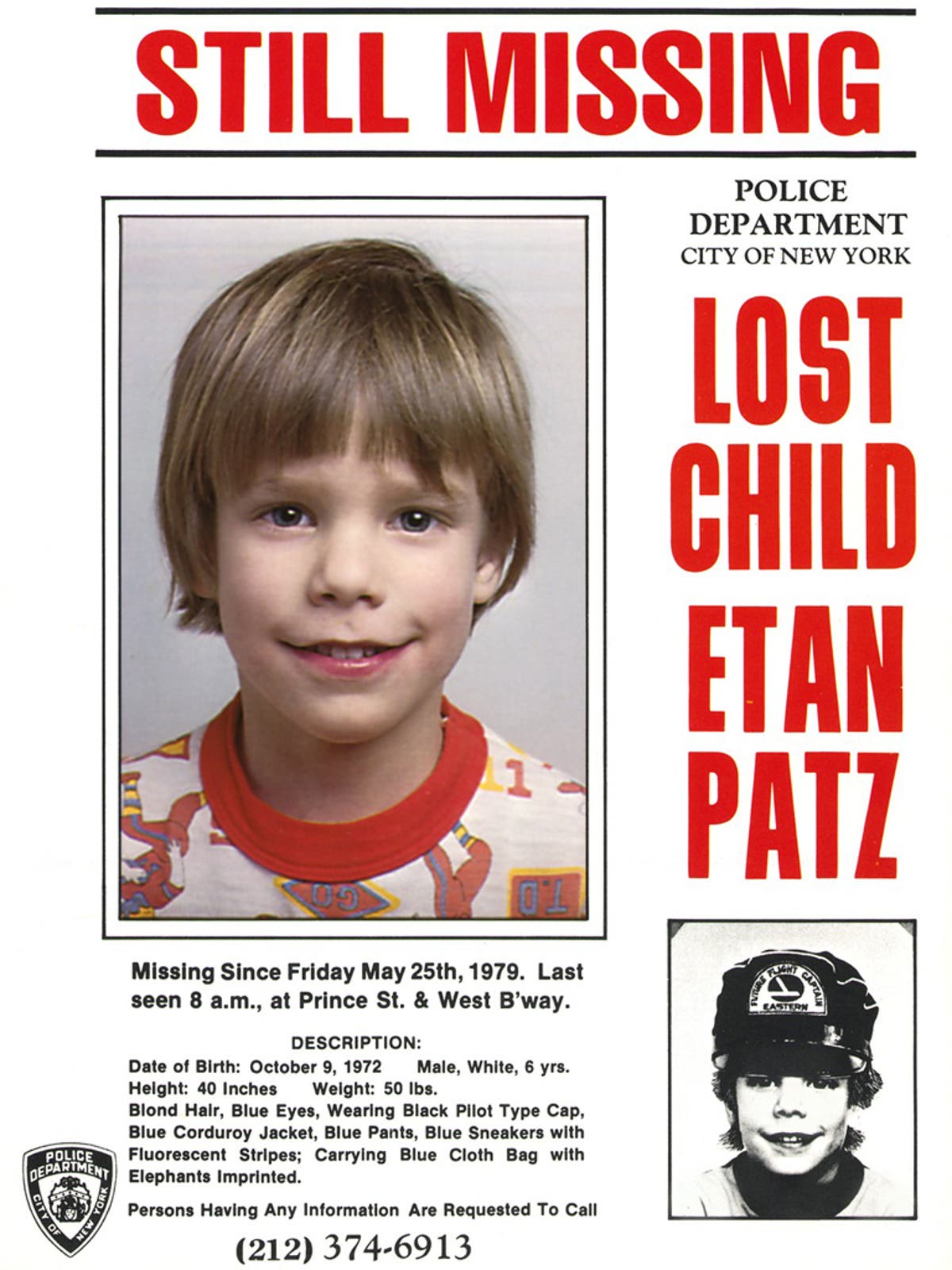This is a detailed description of a missing child poster with a white background. Dominating the left side of the poster is a large, color photograph of a young Caucasian boy, likely around six or seven years old. He has short light brown or blonde hair with bangs and possibly blue eyes. He is smiling towards the camera and is dressed in a white shirt with a red neckband and a design that might represent sports figures. 

At the top of the poster, in bold red capital letters flanked by black lines, it reads "STILL MISSING." Below this, in black lettering, it lists "Police Department, City of New York." In prominent red capitals beneath the photograph, it states "Lost Child Etan Patz."

Further down, the poster provides crucial information:
- "Missing since Friday, May 25, 1979."
- "Last seen at 8 A.M. at Prince Street and West Broadway."
- "Description: Date of Birth: October 9, 1972. Male, White, 6 years old. Height: 40 inches. Weight: 50 pounds. Blonde hair, Blue eyes. Wearing black pilot-type cap, blue corduroy jacket, blue pants, and blue sneakers with fluorescent stripes. Carrying a blue cloth bag with elephants imprinted."

At the bottom right corner, a small black and white photograph of the boy is also displayed, where he is seen wearing a hat and smiling. The poster concludes with a call to action in black text: "Persons having any information are requested to call (212) 374-6913."